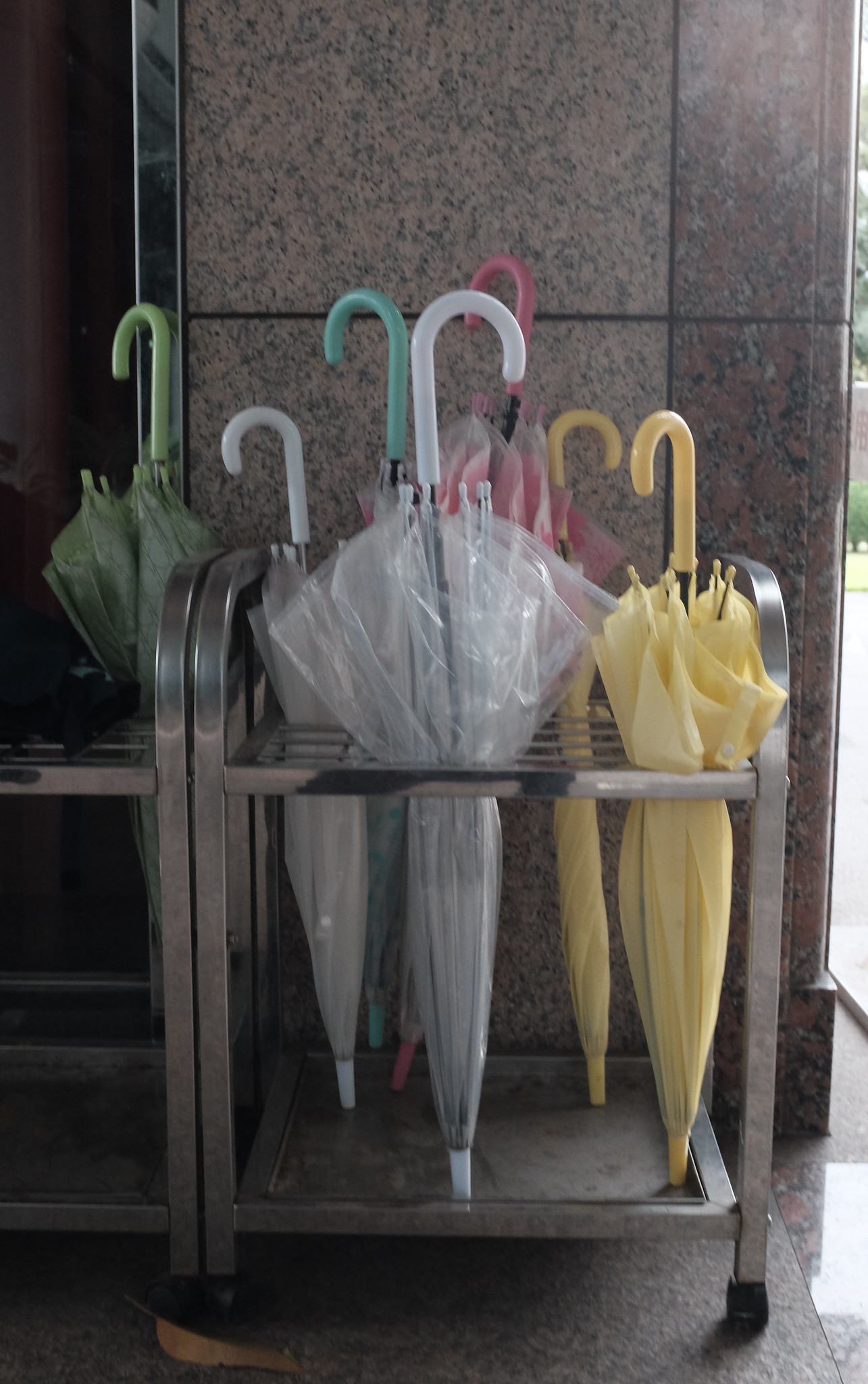The image depicts two custom-made metallic chrome umbrella stands positioned side by side, located against light brown, speckled granite tiles that form both the floor and wall. The interior scene is subtly illuminated by sunlight filtering through a nearby window, casting reflections on the smooth tile surfaces. Each umbrella stand contains multiple collapsed umbrellas held with their curved handles pointing upward. Among the umbrellas are a variety of colors: two light yellow with matching handles, one clear white with a white handle, a pink one, a teal one, a vibrant green one, and another transparent white one. Outside the window, bushes and grass are faintly visible. Additionally, a small brown leaf lies in front of the umbrella stands, adding a natural element to the meticulously maintained indoor space.